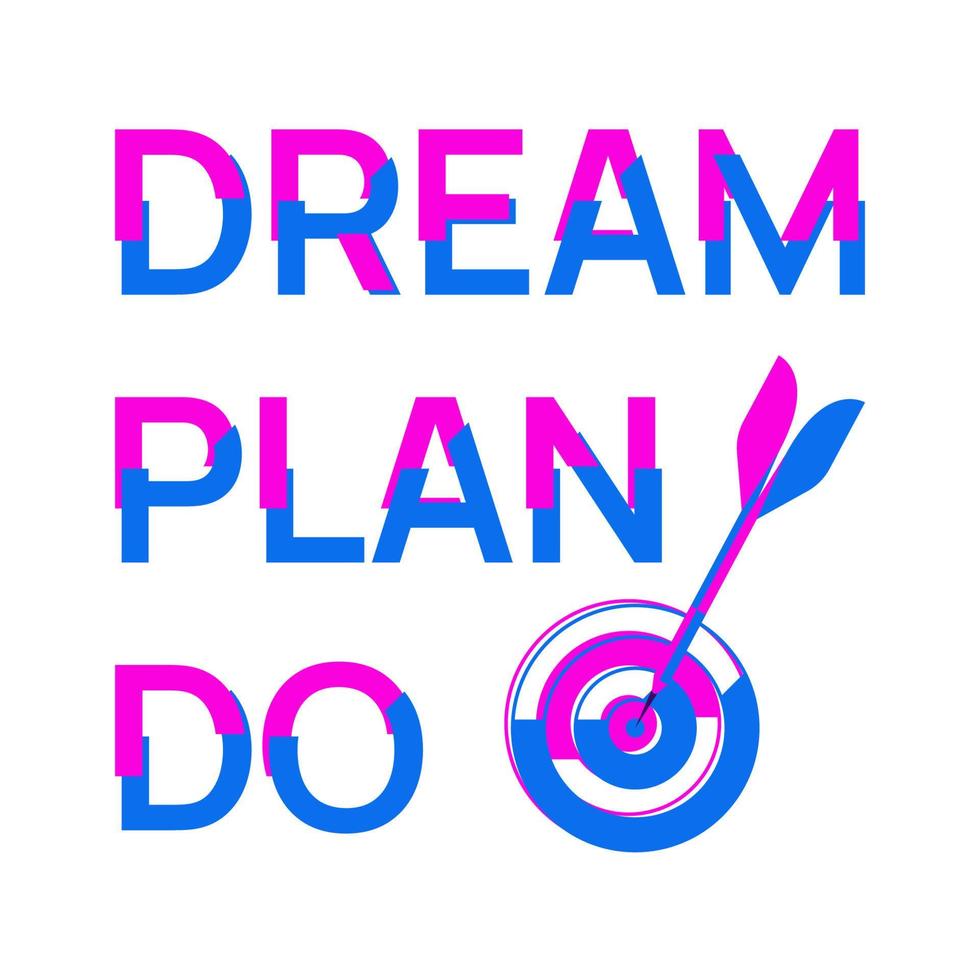The image features a vibrant, handwritten sign on a white background, displaying the motivational phrase "DREAM PLAN DO" arranged vertically from top to bottom. The letters in each word are split into two colors: a vivid hot pink for the top halves and a cool blue for the bottom halves. To the right of the text, there is a detailed illustration of a target, designed with concentric circles in blue, white, and pink. At the center of the target lies a solid blue bullseye, with a dart piercing directly through it. The dart itself is colored half blue and half pink, matching the color scheme of the text. The overall effect is dynamic and eye-catching, potentially serving as a logo or motivational emblem that could appeal to both children and adults, possibly indicating an organization focused on inspiration, consulting, or volunteer work.